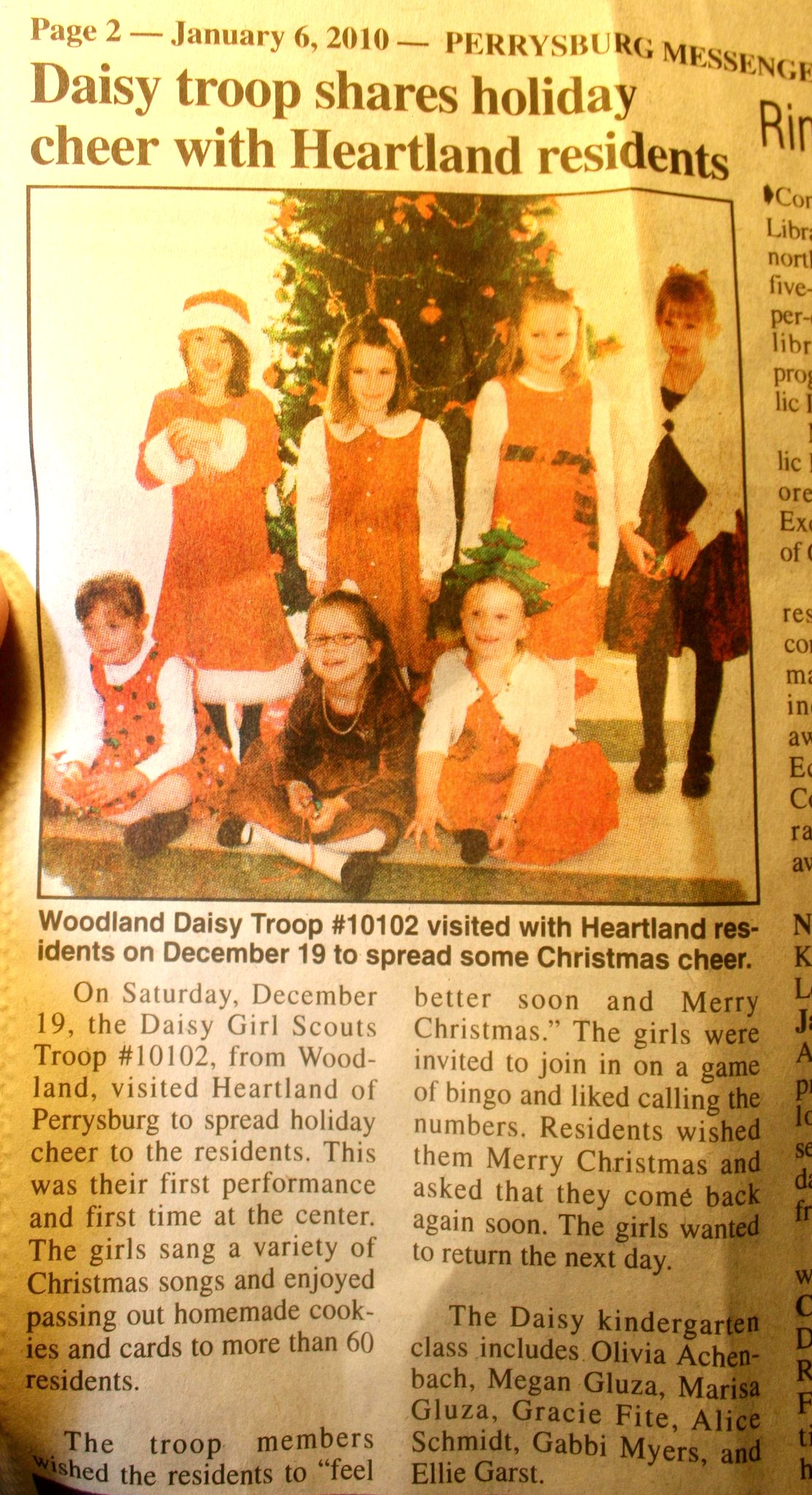The image depicts a yellowed newspaper clipping from the Perrysburg Messenger, dated January 6, 2010, on page 2. The headline above the photo reads, "Daisy Troop Shares Holiday Cheer with Heartland Residents." The photograph shows seven young girls, likely kindergarten age, from the Woodland Daisy Troop 10102. They are gathered around a Christmas tree, with four girls standing in the back and three sitting in front. Most of the girls are wearing festive red dresses, and one is adorned in a Santa hat while another sports a green Christmas tree headband. A few details differentiate them: one girl is wearing a burgundy dress and white cardigan, and another has on a white dress with black dots. Below the photo, the caption states, "Woodland Daisy Troop 10102 visited Heartland residents on December 19th to spread some Christmas cheer." The accompanying article details their visit, noting that the troop sang Christmas songs, handed out homemade cookies and cards to over 60 residents, participated in a game of bingo, and expressed a strong desire to return. The girls, identified as Olivia Atchinsbach, Megan Gluza, Marissa Gluza, Gracie Fite, Alice Schmidt, Gabby Myers, and Ellie Garst, brought holiday joy and left a memorable impression on the residents.